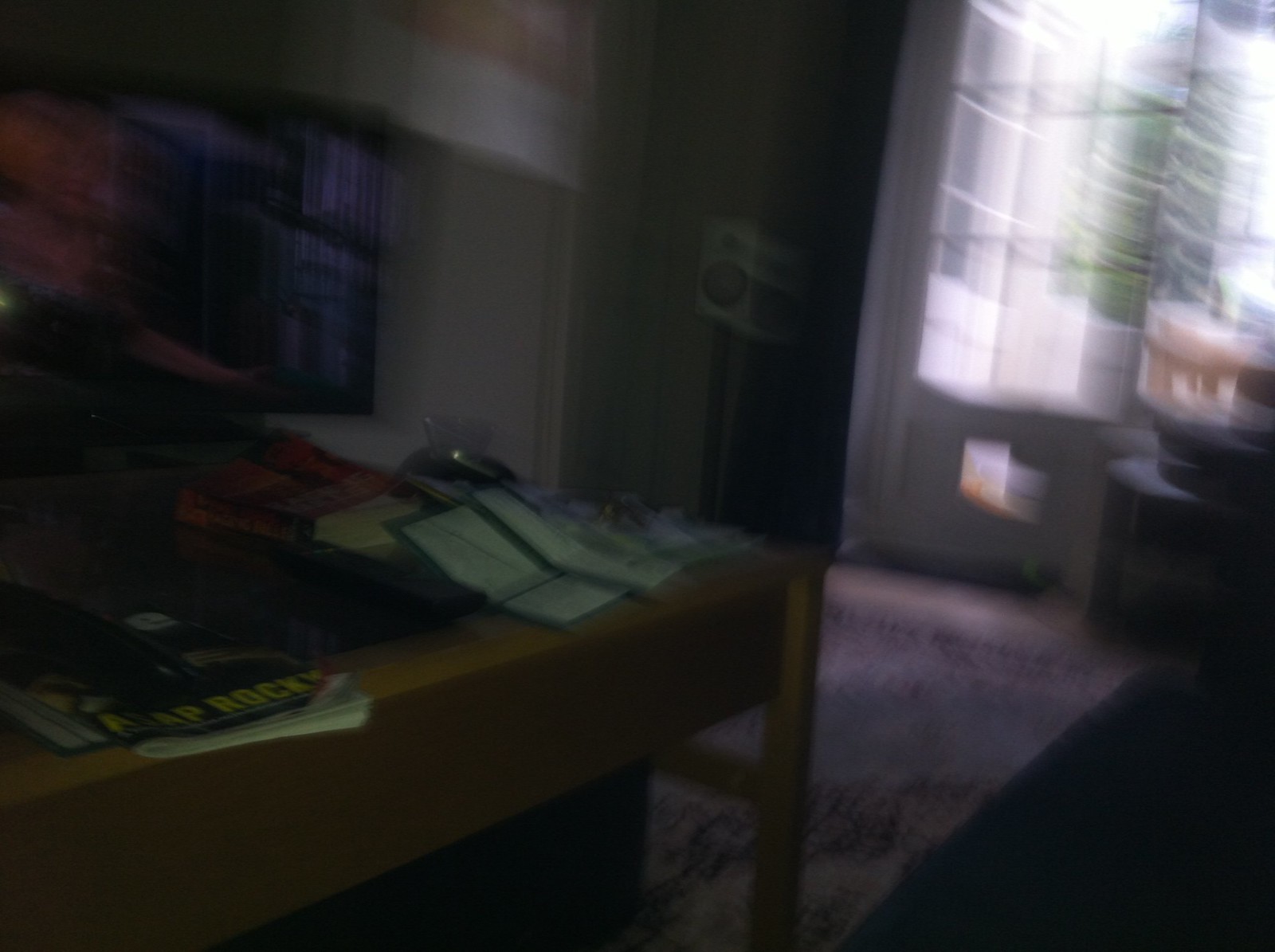A blurry photograph captures the interior of a cluttered home office. On the left side of the image stands a wooden desk, heavily laden with an assortment of books and magazines. Notably, one magazine with a black background prominently features "ASAP Rocky" in bold yellow text. The floor is adorned with a rug showcasing a red and white design. In the back corner, a white speaker perches atop a black pole. To the right, natural light filters in through a window framed by white curtains, revealing a tree outside. Despite the overall blurriness and distortion, the cozy, lived-in ambiance of the room is evident.